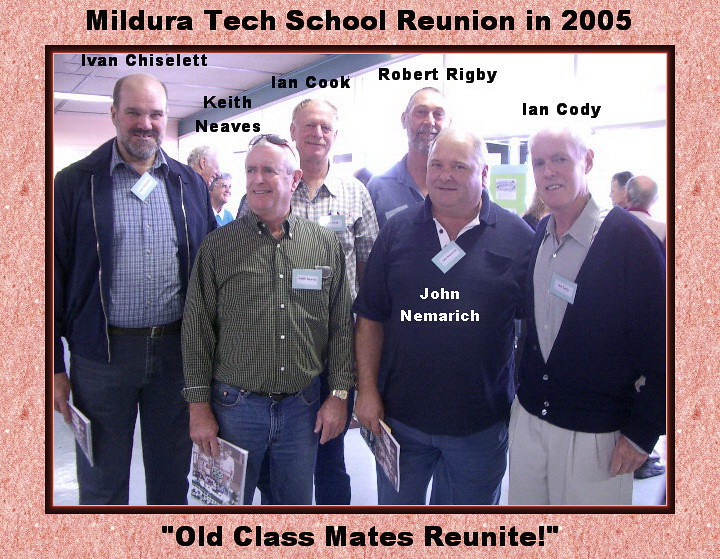This photograph captures a heartwarming moment from the Midder Tech School Reunion in 2005. Posing for the camera, a group of six men stands together, four in the front and two in the rear, all smiling warmly. Above the men, who are identified by their names written on the photograph, the caption reads "Midder Tech School Reunion 2005, Oklahoma Students Reunite." The men are casually dressed in a mix of t-shirts and jackets, with some wearing jeans and others in khakis. Badges and programs in hand, they stand in what appears to be the lobby, as ceiling tiles and light streaming in suggest an indoor setting. Each man exudes a nostalgic excitement, celebrating their reunion and the shared camaraderie of old classmates. The photograph is bordered by a pink frame, giving it a postcard-like appearance, capturing not just the faces but the joyful essence of reconnecting with old friends.